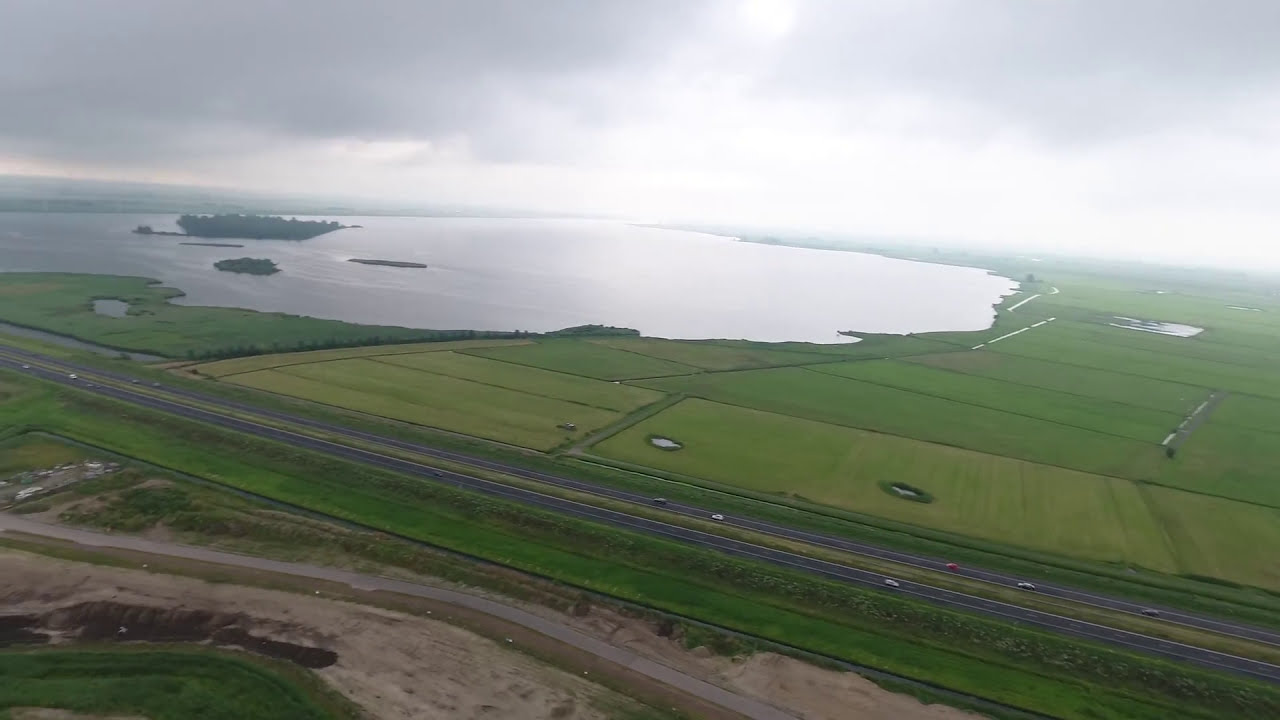This aerial photograph captures a sprawling landscape composed of diverse elements. Dominating the left side of the image is a large, silver-hued lake, with an island of trees nestled in its midst. Overhead, the sky is overcast with gray clouds, partially veiling the sun, contributing to a muted light that bathes the scene in subdued colors.

Centrally positioned and towards the right, vast green fields stretch out, suggesting fertile farmlands that add a vibrant contrast to the silvery water. A prominent feature cutting through this pastoral expanse is a dark, four-lane highway lined with vehicles traveling in both directions, highlighting human activity within this natural setting. 

Near the highway, there are patches of green grass and possibly a dirt road, adding texture and variety to the landscape. The image is devoid of buildings and text, emphasizing the predominance of natural and rural elements. The palette includes earth tones—rich greens, browns, and grays—complemented by the reflective silver of the lake and the muted tones of an overcast sky, creating a serene yet dynamic aerial vista.